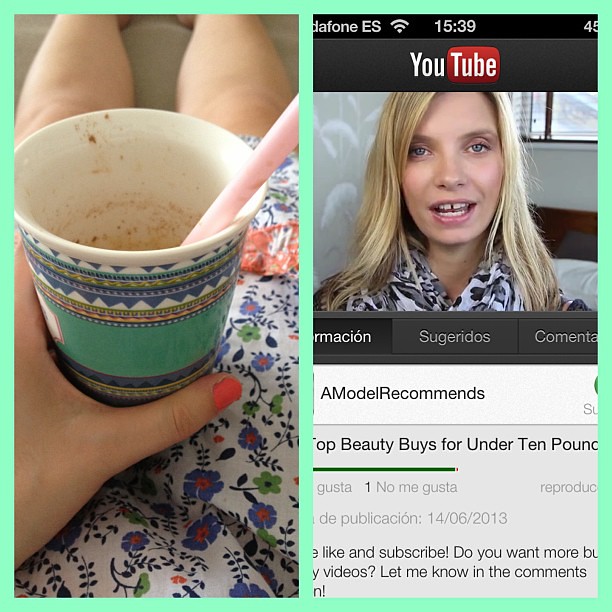The image is a large, square frame, segmented with a light green, Eastern green border dividing it into distinct parts. On the left side, there is a vertical rectangular section showing a young woman, lying down with her legs visible. She is dressed in a white floral dress adorned with blue flowers. Her left thumb, painted with light pink nail polish, is holding a brown paper cup decorated with a pattern of teal, medium blue, yellow, and white designs. The cup, which contains remnants of brown substance—possibly ice cream—and has a straw sticking out from it, rests on her stomach area.

On the right side of the image, a cropped segment of a YouTube page is visible. At the top of this section, the YouTube logo appears above the face of the young woman previously described. She has long, straight blonde hair and is wearing a top with a gray, black, and white cheetah print pattern. She has a noticeable gap between her top front teeth. A window and a wall are in the background. The timestamp at the very top reads 15:39, alongside a Wi-Fi symbol, suggesting it was captured from a cell phone. At the bottom, there is text instructing viewers to "subscribe" and "let me know in the comments section," indicating this image is promoting a YouTube video.